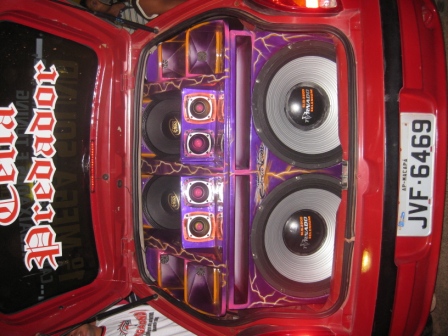This photograph, oriented sideways requiring you to tilt your head to the left for proper viewing, captures the trunk of a shiny red car, which houses an elaborate sound system. At the bottom right, a white license plate reads "JVF-6469." The interior of the trunk door features a medieval-style decal with the word "Predador" (P-R-E-D-A-D-O-R) prominently visible. The sound system itself dominates the trunk, presenting a cohesive purple and orange lightning motif. In the forefront are two enormous subwoofers with black centers and silver surrounds, encased in purple boxes. Above them, two smaller sets of speakers share the same decorative theme, while two larger speakers are positioned at the very top, aligned wider than the smaller sets beneath them. The arrangement indicates a well-constructed and visually striking audio installation designed to impress.